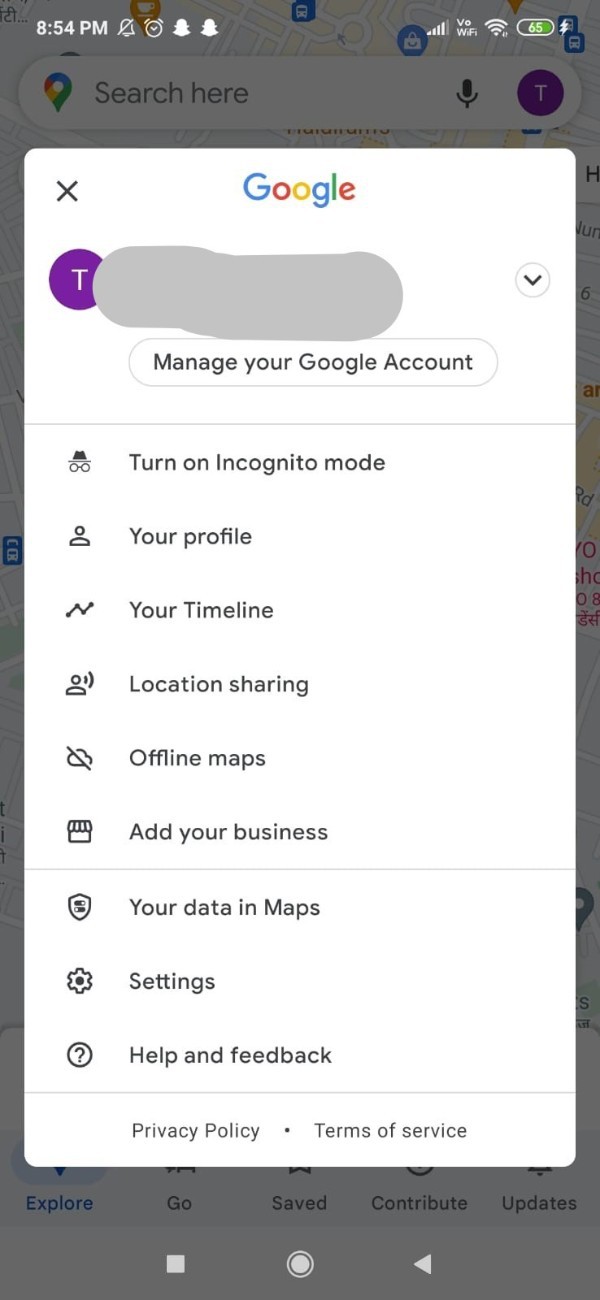The image captures a mobile device screen at 8:54 p.m. The upper-left corner displays the current time of 8:54 p.m., accompanied by several notification icons—including Snapchat, an alarm, and muted notifications. On the upper-right, the battery is at 65%, with indicators for both cellular signal and Wi-Fi connectivity. Below, the background showcases a Google search bar with a location icon in Google colors and a purple circle containing a white 'T' to the right.

Prominently centered on the screen is a Google pop-up window. At the top of this window is a black 'X' in the upper-left corner for dismissal. Below the 'X,' the purple circle with the white 'T' reappears beside blurred-out account information. The pop-up menu lists several options: "Manage your account," "Turn on Incognito mode," "Your profile," "Your timeline," "Location sharing," "Offline maps," "Add your business," "Your data in Maps," "Settings," and "Help and feedback." Under these options is a thin, horizontal gray line. At the very bottom, "Privacy Policy" and "Terms of Service" are listed with a small black dot positioned between them.